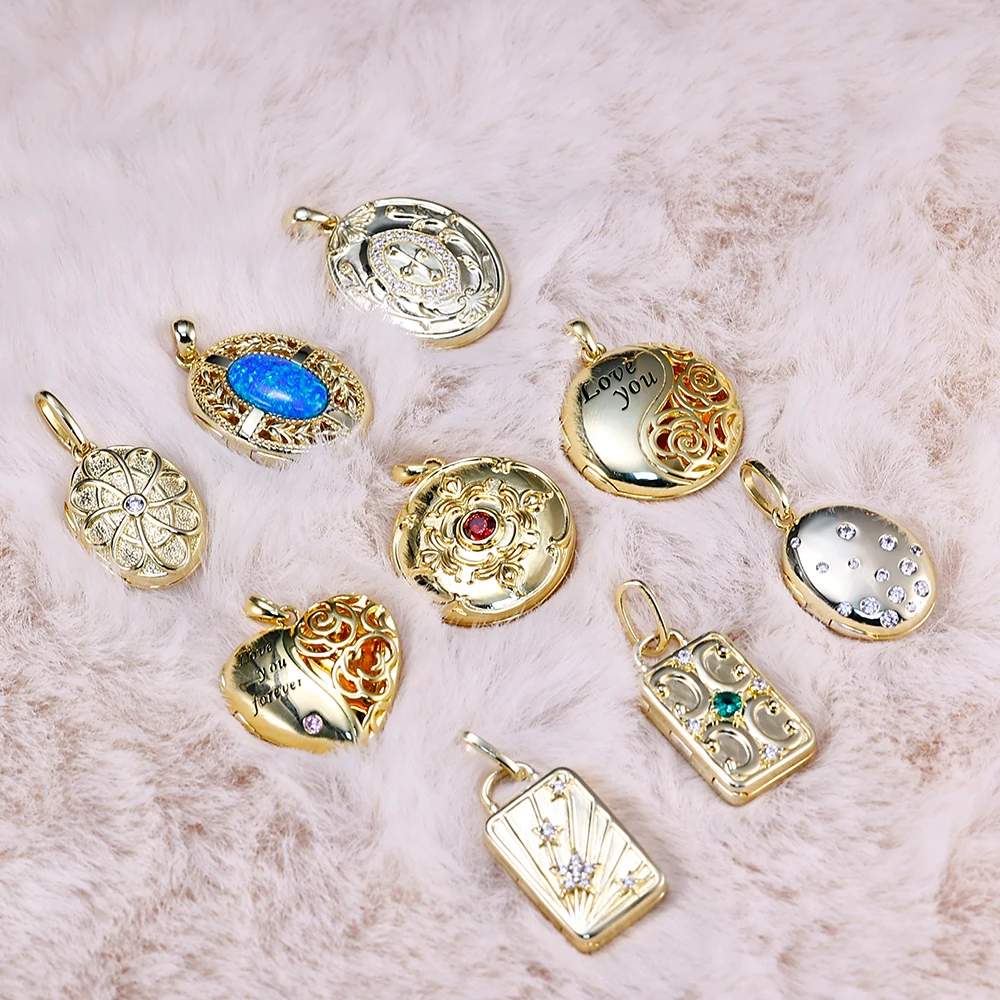This indoor photograph features nine distinct metal pendants, possibly customizable jewelry for sale, arranged in three rows on a plush, fuzzy blanket with a white and pinkish hue. These pendants, predominantly gold or silver, are of various shapes: four ovals, two circles, two tall rectangles, and one heart. Notably, the heart-shaped pendant has the inscription "Love You Forever" and includes a purple stone. Among the pendants, two rectangular ones are on the bottom left, with one featuring a green gemstone, while one circular pendant has a red gemstone, and an oval pendant showcases a blue gemstone. Many of these charms contain clasps, indicating they could be attached to necklaces or bracelets.